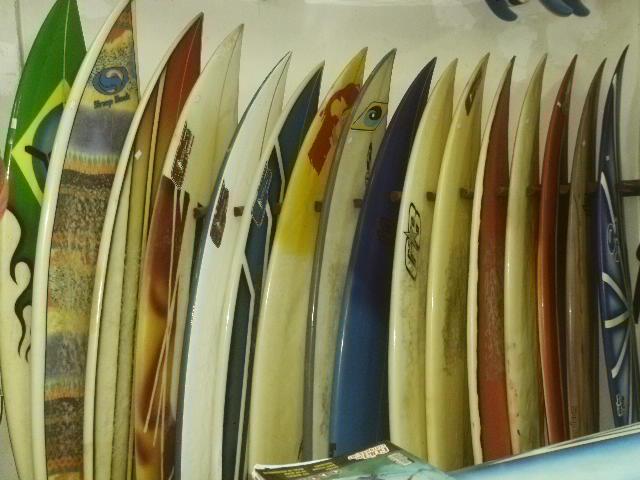The image showcases a vibrant, organized display of surfboards, all standing upright against a white wall. The surfboards vary in colors, including green, beige, yellow, red, and occasionally feature decorative elements like yellow diamonds or eye motifs at their tips. These boards are stacked neatly, separated by wooden pegs that protrude from the wall, preventing them from toppling over like dominoes. A closer look reveals fine details such as a wooden rack structure and patches on the white wall behind the surfboards. In the top right corner, something blue hangs off the wall, partially cropped out of view. On the bottom left corner, there is a light blue surface, possibly a table, on which a partially visible magazine or book with a black, teal, red, and yellow cover lies. This setting appears to be a place where one can either buy or rent surfboards, selecting from a variety of sizes and colors.